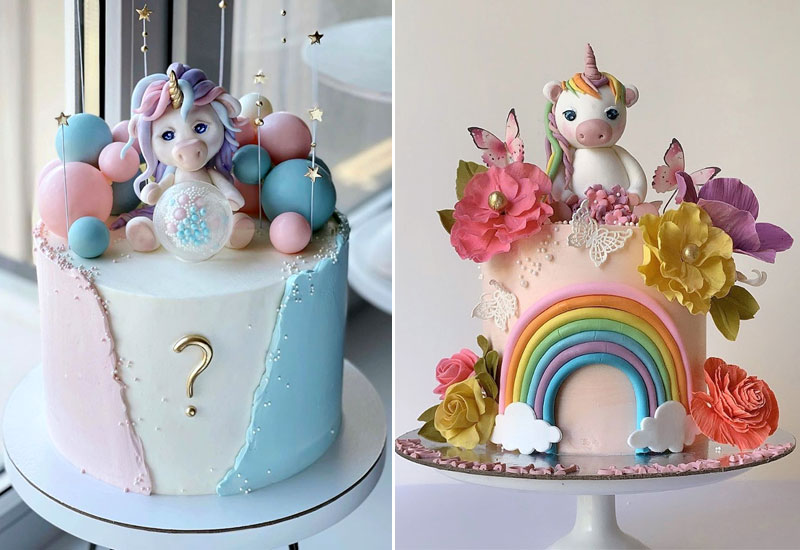In this image, there are two custom-made, round, single-layer unicorn cakes displayed side-by-side, separated by a thin white line. Both cakes are on cake stands and set in a kitchen with other trays visible in the background.

The cake on the left features a pastel color scheme. The sides are decorated with light pink and blue fondant on either side of a central white section that bears a gold question mark, suggesting a gender reveal theme. The top of the cake is adorned with a unicorn figurine with pink and blue hair, a gold horn, and is surrounded by pink and blue balls. There are also sprinkled white pearls and gold-star-topped sticks adding to the decoration.

The cake on the right is decorated in more vibrant colors. It is primarily pale pink and features a large rainbow on the front, with clouds at either end. This cake also has a unicorn on top, with a colorful mane of orange, pink, yellow, green, and purple, and a purple horn. Additional decorations include flowers with gold centers and a variety of colors (pink, yellow, purple), two white lace-like butterflies, and smaller pink and purple flowers. The cake stand is also adorned with coral-colored, pink, and yellow flowers.

Overall, both cakes are intricately decorated unicorn-themed desserts, likely made for a celebratory occasion.